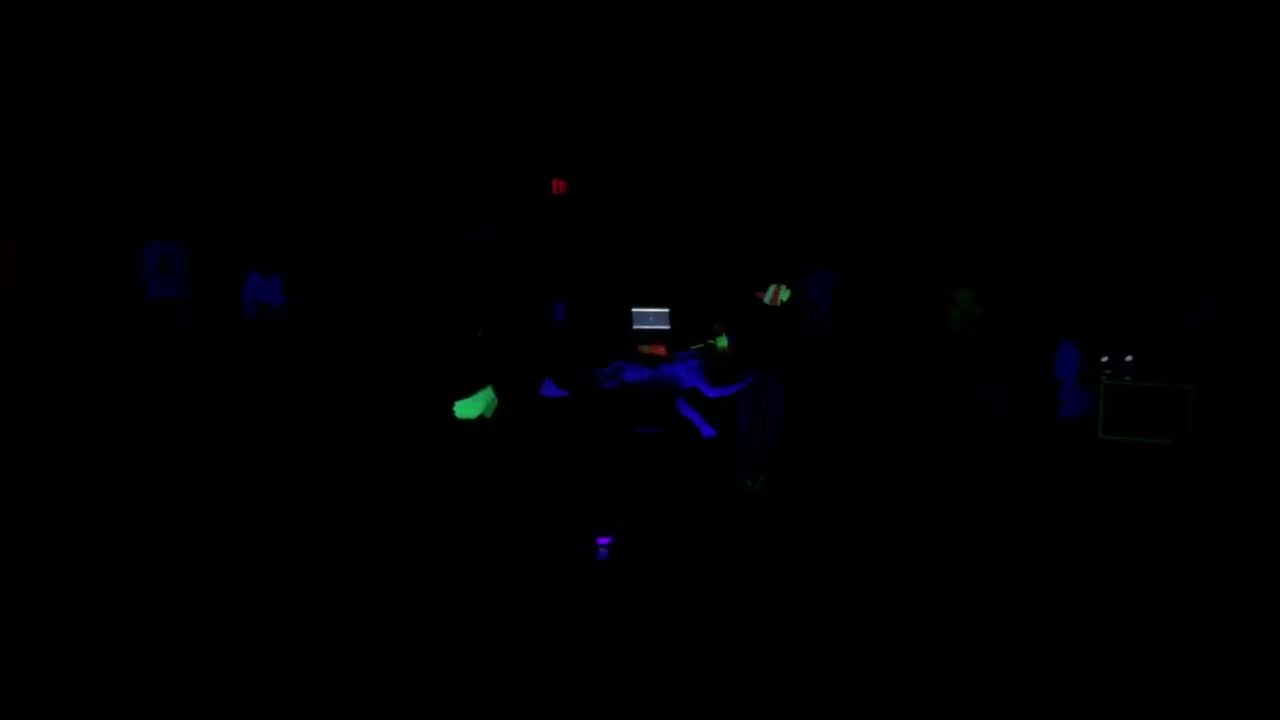In this vividly dark, computer-animated image, the scene is enveloped in near-total darkness, with the dominant visual elements being vibrant, fluorescent blue hues. At the center, a figure, possibly a scuba diver in a blue wetsuit, seems to be moving about in murky waters. The diver appears to be positioned prone and is holding a spherical object in their left hand. Fluorescent green and red accents punctuate the scene; a small green square is visible to the left of the figure, and the far right showcases what seems to be a head, also illuminated in bright blue, facing towards the central figure. The immersive darkness obscures the background, directing all focus on the vivid performers in the forefront. The composition suggests an intriguing blend of underwater exploration and the strikingly theatrical aesthetics reminiscent of the Blue Man Group.